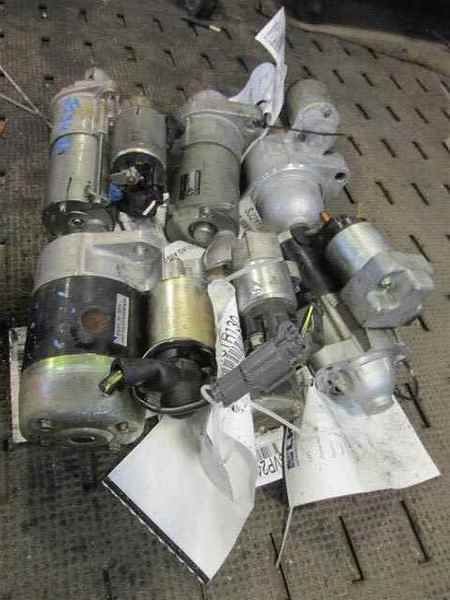This color photograph depicts nine cylindrical metal objects, likely engine parts or small motors, arranged roughly in two overlapping rows on a dirty black rubber mat that appears gray due to the grime. The mat features numerous hollow rectangular slits. Most of the cylinders are silver-colored, with some showing hints of gold and black. These metallic objects, which also display various nuts and bolts, are marked with white tags bearing barcodes or numbers. Some of these tags are visibly tied to the objects. Towards the bottom right of the arrangement, there are two or three sheets of paper, one folded and the others turned upside down, with black text reading "VP2A." The cylinders appear segmented into two or three parts, and some have central components that look designed to be turned.